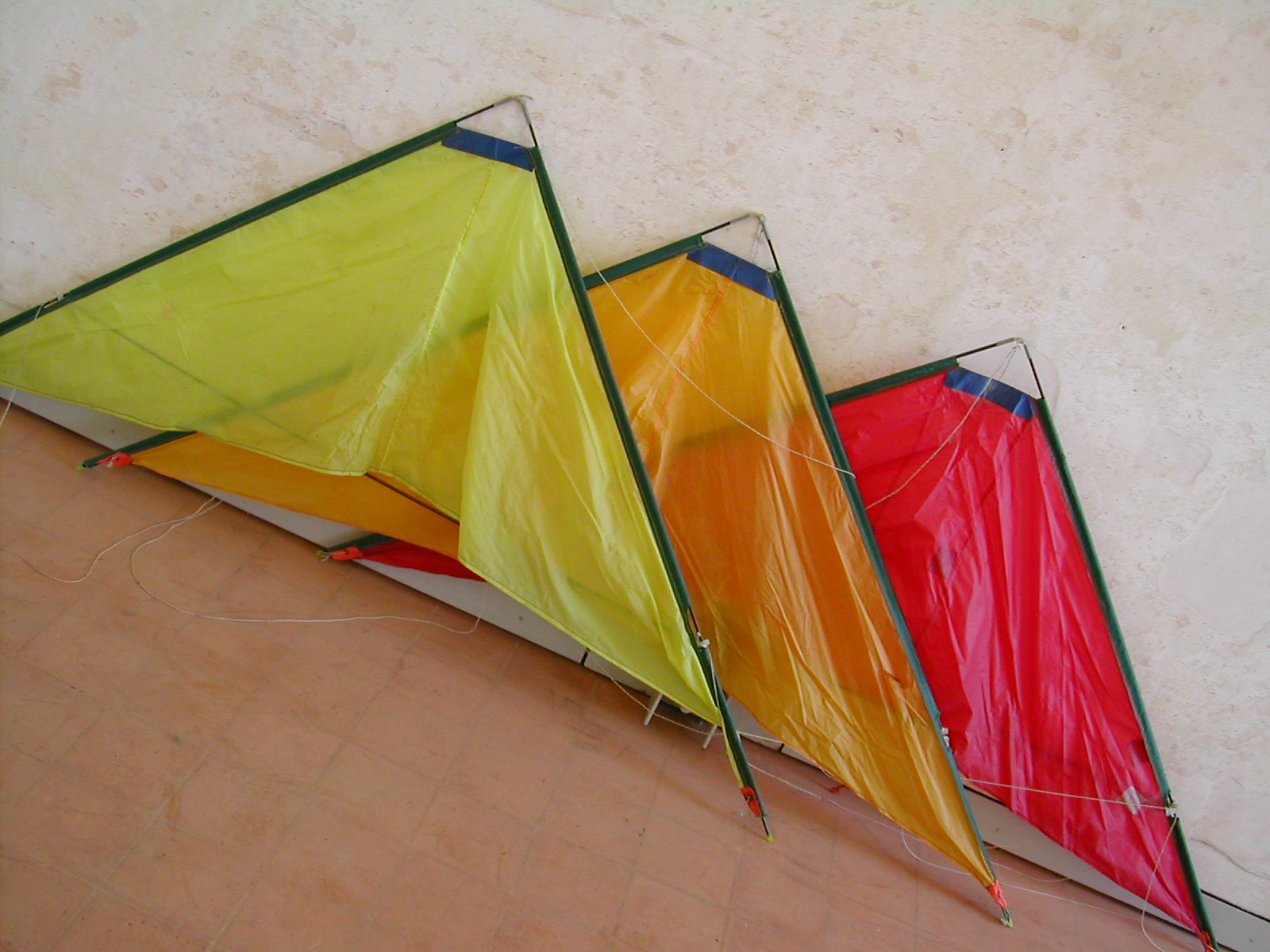This image captures a color photograph taken outdoors with natural lighting. The photograph is slightly tilted to the right, presenting a diagonal view. The background consists of a textured beige or white wall, possibly made of concrete or large bricks, adding a rugged appearance to the scene. 

In the foreground, a light brown or orange-tinted tile floor stretches out, with the tiles arranged in a square pattern. The tiles appear dusty, obscuring any clear view of the grout.

Leaning against the wall are three triangular kites in a cascading arrangement, each slightly overlapping the one behind it. The first kite on the left is a light yellow color, the middle kite is orange, and the last kite to the right is red. Each kite is framed with metal edges and has blue tape forming small triangular tips at the top. Some strings are visible, dangling from the kites.

The details and vibrant colors of the kites stand out prominently against the plain background, creating a striking contrast. The composition and the angle of the photograph provide a unique perspective, making the kites appear like abstract, colorful mountainous shapes against a textured wall.